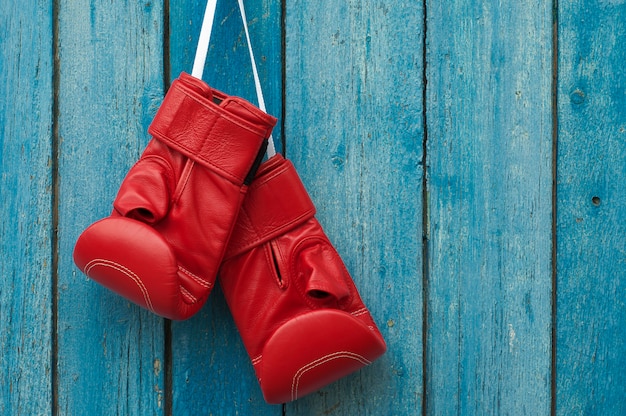A pair of bright red boxing gloves hangs on a distressed, bluish-green wooden fence. The fence, which varies in shades of blue with hints of brown, shows signs of wear and chipping. The boxing gloves are tied together with a white string, creating a striking contrast against the rustic background. The gloves, appearing brand new, feature mitten-style finger compartments with an open thumb design. They are securely attached to the fence via a hook or nail, though the exact attachment point is obscured.